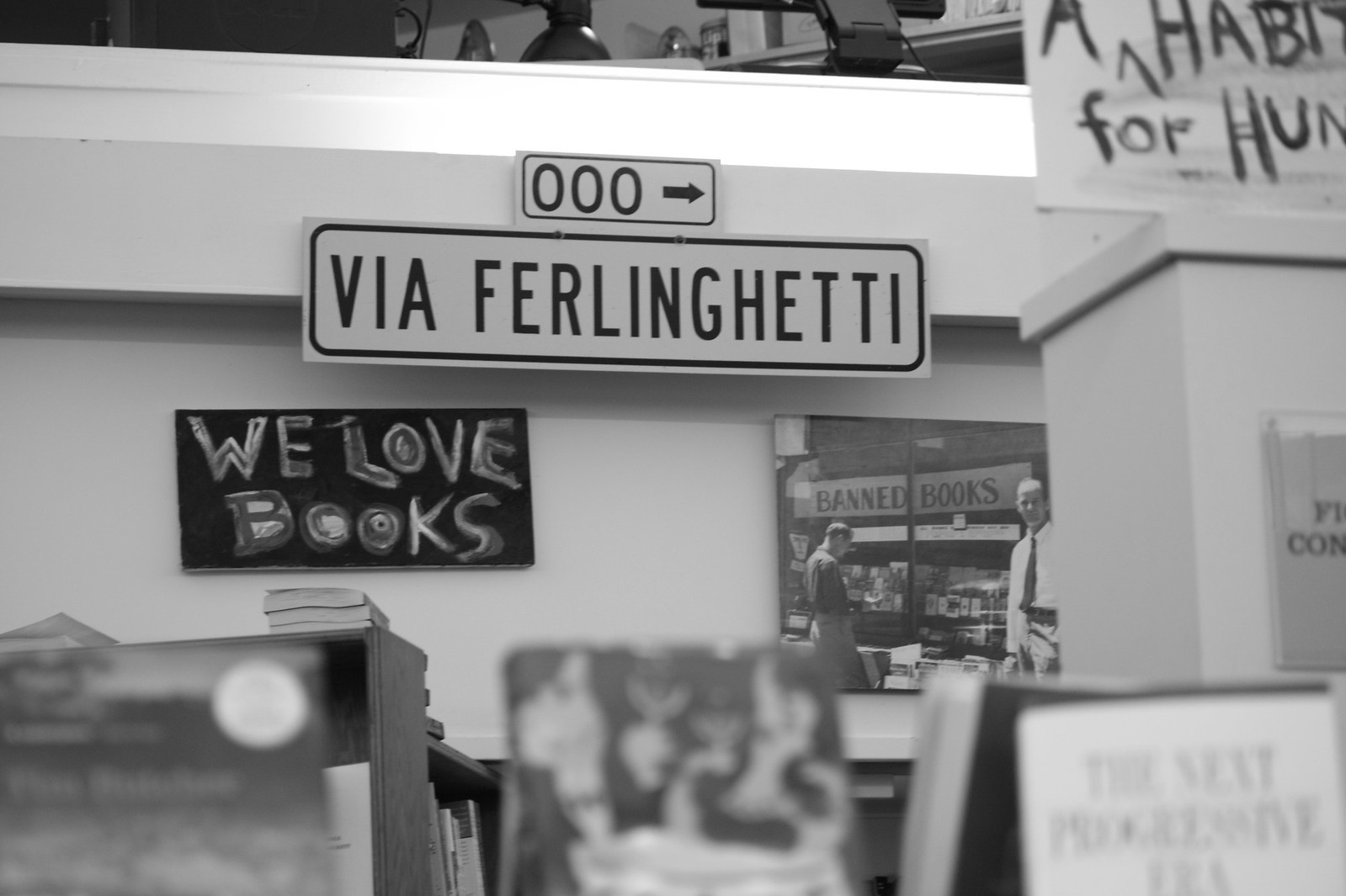In this black and white image, the focus is on a wall adorned with various signs and posters, suggesting a possible bookstore or community space. Central to the composition is a street sign reading “Via Ferlinghetti” (F-E-R-L-I-N-G-H-E-T-T-I), displayed prominently within a black rectangle with rounded edges. Just above this, another sign—also within a rectangular frame—features “000” and an arrow pointing to the right.

Directly beneath the street sign is a handmade sign that reads “We Love Books,” created with what appears to be gray pencil or pastel, lending a textured, artisanal feel to the artwork. To the side of this sign, there’s a picture featuring the words “Banned Books,” possibly depicting two individuals standing near a library or a similar environment.

The scene includes additional elements visible around the main signs: various handmade posters and different pictures, along with several books resting on a shelf, contributing to the cluttered yet cozy aesthetic of the space. The white wall serves as the backdrop, making the black and white signs stand out even more.